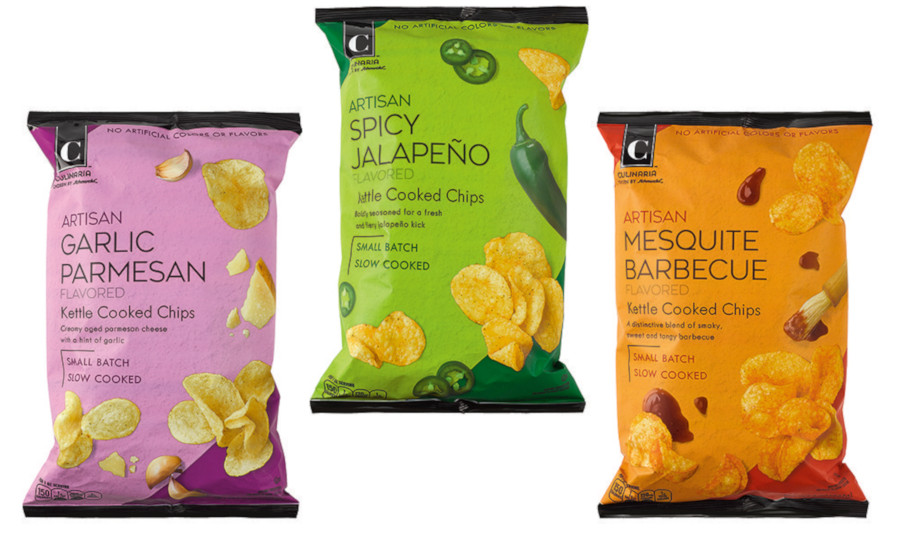The image displays three bags of Artisan kettle-cooked potato chips arranged against a white background. On the left, the bag is primarily light purple with darker purple accents and features images of plain potato chips. The text on the bag reads "Artisan Garlic Parmesan Flavored Kettle Cooked Chips," emphasizing that they are "small batch, slow cooked" with "aged parmesan cheese and a hint of garlic." 

In the middle, the bag is green with lighter and darker shades and showcases golden-colored chips alongside images of whole and sliced jalapenos. The text describes these as "Artisan Spicy Jalapeno Flavored Kettle Cooked Chips," offering "a fresh jalapeno kick" and highlighting the same "small batch, slow cooked" process.

On the right, the bag is predominantly light orange with darker orange sections. It shows orange-hued chips with a brush of barbecue sauce and splashes of sauce imagery. The writing identifies these as "Artisan Mesquite Barbecue Flavored Kettle Cooked Chips," noted for their "distinctive blend of smoky, sweet, and tangy barbecue flavors," and also mentions they are "small batch, slow cooked."